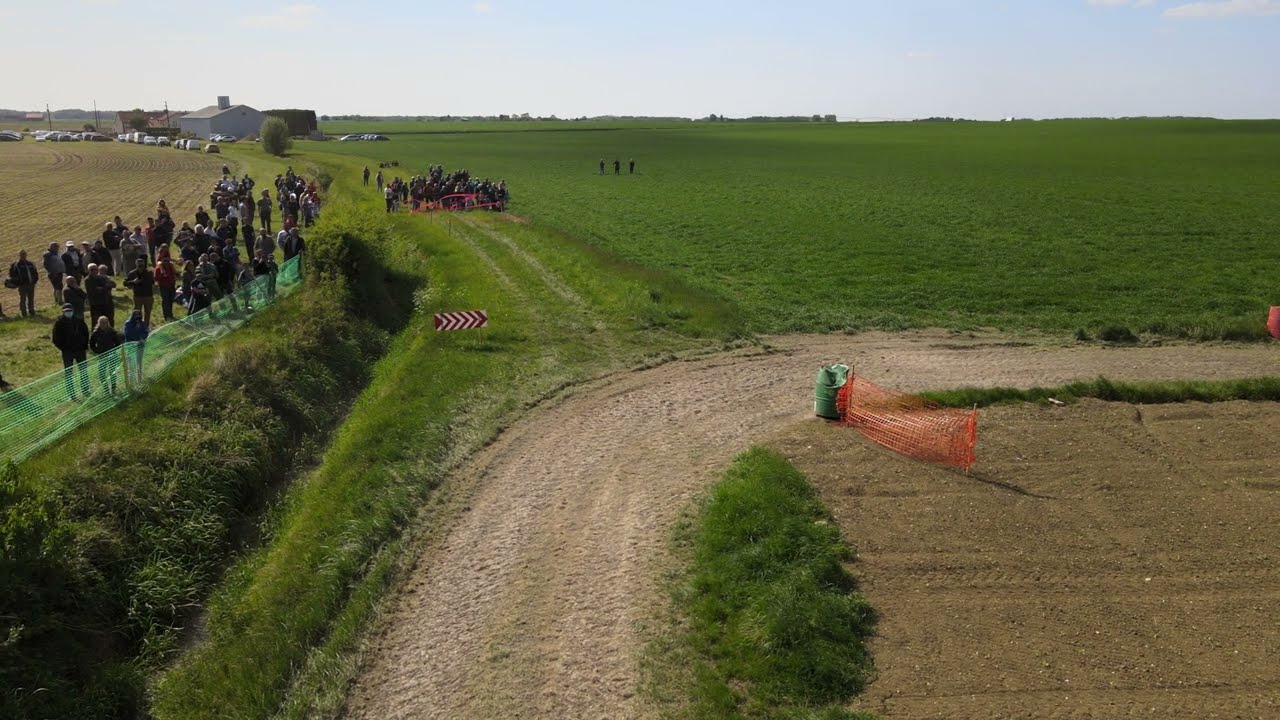The photograph captures a vibrant outdoor daytime scene in a sprawling, flat field punctuated by various elements. Central to the image is a dirt road that begins at the bottom center and sweeps right in a curving arc, forming a semi-circle. To the left of this dirt road, an embankment, seemingly elevated slightly, is populated by a crowd of approximately 100 people. This group is cordoned off by a green mesh fence at the top of a grassy knoll. Adjacent to this group, in the lower right corner of the field, another 100 people are gathered behind a red tape barrier that appears improvised.

In the foreground on the right, the road transitions from brown dirt to greener pastures, marked by a red and white arrow sign pointing right. Below this sign, a green barrel supports an orange plastic fence post, hinting at further makeshift divisions. In the far background, three isolated individuals stand equidistant from each other, staring towards the camera from about 25 feet away, their presence more distinct than a cluster of parked cars further behind.

Adding to the scene’s texture, a piece of farm equipment, perhaps in use for mowing, is noted amidst the clusters of people, suggesting an agricultural backdrop. The blue sky, dotted with a few clouds, envelops the entire scene, accentuating the picturesque and busy communal gathering in this expansive field.